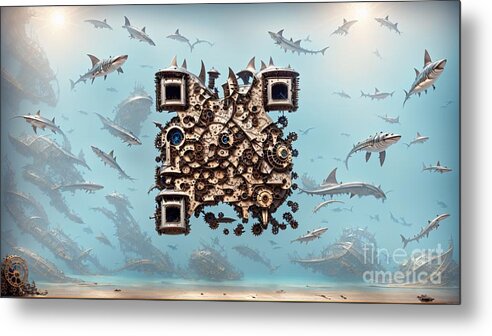This artistic painting, featuring the watermark "Fine Art America" in the lower right corner, presents a captivating underwater scene bathed in light from above. The light sources appear like ethereal sunbursts on both the top right and left, illuminating the entire image. Throughout the painting, sharks of varying sizes swim with an otherworldly appearance due to additional fins on their top and bottom. These sharks navigate a blue ocean backdrop filled with intricate underwater life and shipwreck remnants that fade into the murky depths at the bottom.

Prominently in the center, an irregular pattern in browns and golds, reminiscent of a mechanical or QR code-like design, captures attention. This pattern has distinct blocks in three corners, surrounded by variously sized spots. On closer inspection, it evokes a sense of enigmatic digital symbolism. The ocean floor in the bottom left corner houses shells and possibly a snail, adding to the rich detail of this intriguing underwater ecosystem.